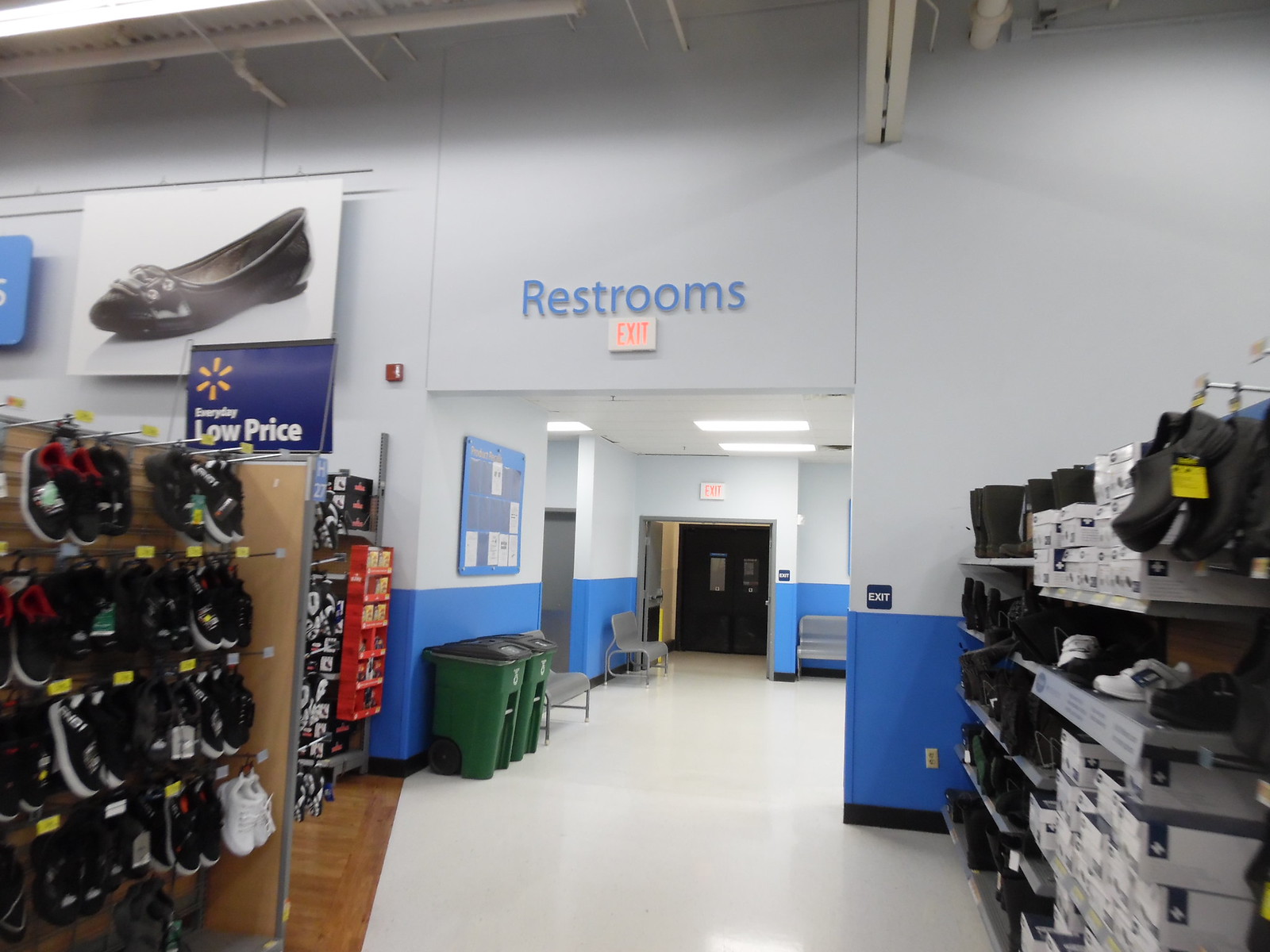This image captures a section of a Walmart store. The floor is a pristine white, and to the left, there's a display shelf adorned with multiple pairs of black shoes, each marked with bright yellow price stickers. On the right side of the image, there's a stacked arrangement of shoe boxes in various colors, topped with some shoes on display. Additionally, some black shoes are hanging with yellow price tags attached.

In the background, there's a white square signage featuring red text, likely providing some store information or promotion, alongside blue lettering that directs to the "Restrooms." The top left of the image shows another white square, also featuring a black shoe and red lines framing it. Centrally located, there's a white square which could be part of the store’s promotional material, and at the bottom of the image, there's a glimpse of green waste bins, gray chairs, and a magazine, possibly indicating a nearby seating or rest area in the store.